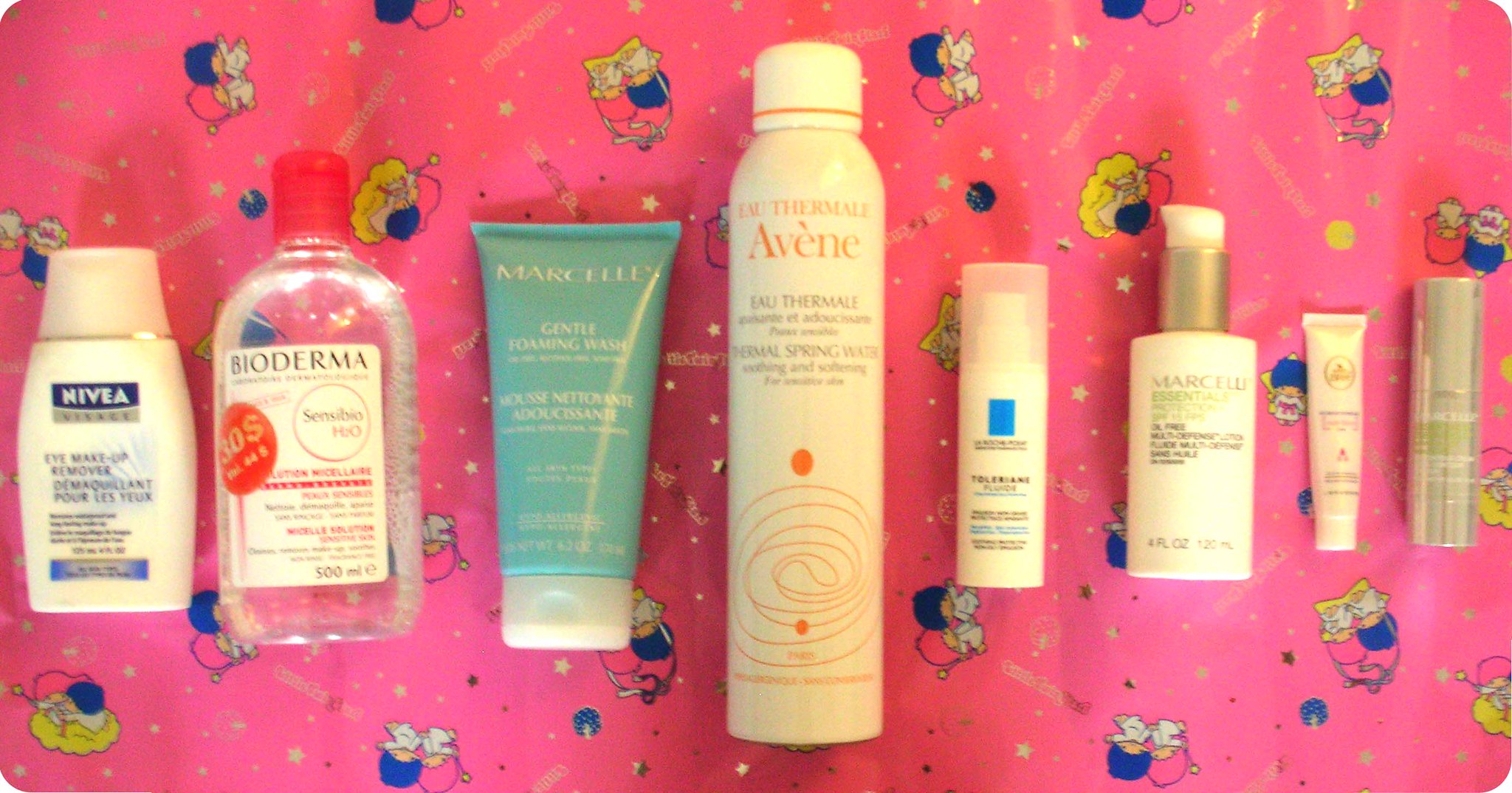A vibrant, landscape-format photograph features eight assorted cosmetic products, meticulously arranged from left to right on a pink background adorned with playful illustrations of cartoon children and stars. Captured from a bird's-eye perspective, the products are laid flat on what appears to be a placemat. Each item represents a different brand, including Nivea, Bioderma, Marcel's, and Avene, with a few others indistinguishable due to slight blurriness in the image. The selection includes diverse shapes and sizes, showcasing items such as eye makeup remover and foaming wash. The whimsical background contrasts with the structured alignment of the cosmetics, highlighting the variety in both design and function of the beauty essentials.